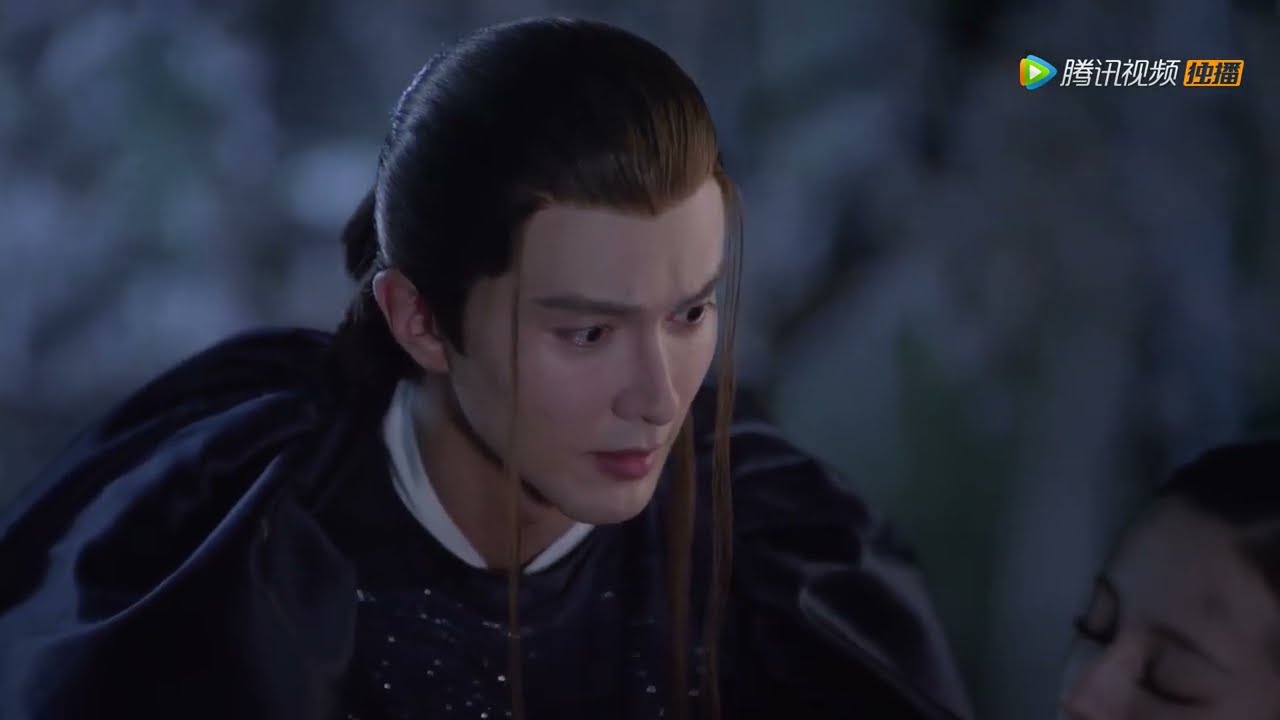The image appears to be a detailed still from a Japanese fantasy television show or video game, featuring a young Asian man in his early 20s. He has a pale complexion and intricate hairstyle: his hair is neatly pinned back with long, brown strands framing his face. He wears a black, puffy robe or coat with a white collar detail, and his expression is one of sadness or concern. The scene is dimly lit, potentially illuminated by moonlight, with a blurred gray background, enhancing the focus on the characters. In the lower right corner, there is a partially visible woman with closed eyes and brown hair. The upper right of the image features Asian characters, possibly a logo or title of the show or game, along with a play button and additional text in various colors including green, red, and yellow.